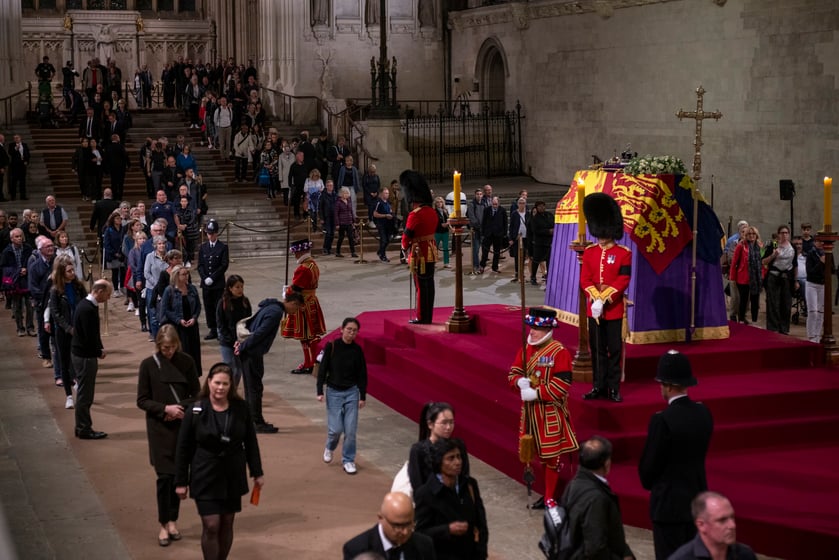The photograph captures a solemn scene inside a large, cathedral-like space, possibly marking a significant ceremonial event, such as a royal funeral. Central to the image is a red-carpeted platform, elevated and framed by carpeted steps, adorned with tall candles and a cross standing prominently at its near side. Atop the platform rests a coffin, draped in a majestic ensemble of red, gold, and black, with an ornate covering of purple and yellow hues. Floral tributes lay upon the coffin, adding to the poignant display of respect.

Flanking the coffin, two English soldiers stand vigil, dressed in traditional red coats, black pants, and tall black bearskin hats, embodying historical symbolism and honor. Additional guards and police officers surround the area, ensuring a dignified atmosphere.

In the foreground, beyond the platform, several people are visible, some walking, while others stand and bow, paying their respects. To the left, a grand staircase descends, with velvet ropes guiding the procession of individuals forming orderly lines as they approach or leave the platform. The surrounding walls and floor feature a palette of green, grey, and brown, enhancing the overall solemnity and reverence of the space. The detailed and elaborate setting suggests the mourning of someone of considerable importance, possibly royalty, hinting at the presence of a significant figure like Queen Elizabeth.